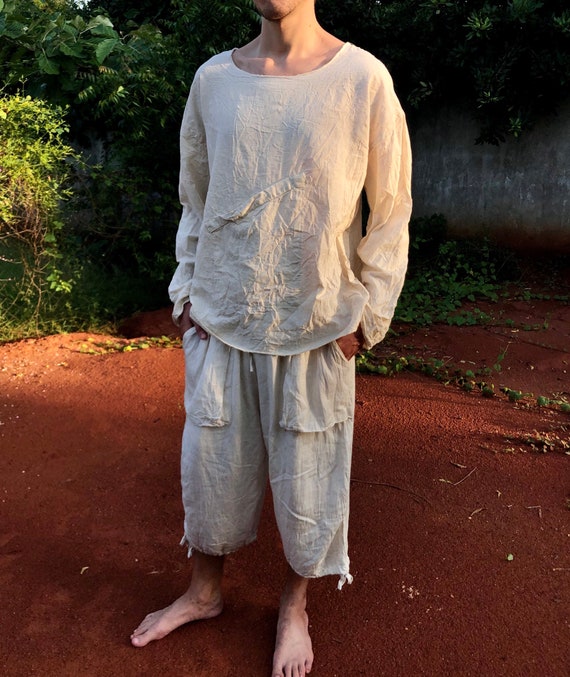The photograph showcases a young man standing barefoot on a flat, reddish-brown dirt surface. The man is only visible from his feet up to his chin, with the top part of his head out of frame. He is dressed in white, cotton-looking pants that end around mid-thigh and feature large pockets on the front. His hands are tucked into these pockets, and he is wearing a long-sleeved shirt made of a similar, heavily wrinkled material with a low scooping neckline. In the background, there is lush green vegetation, including ferns and trees, while the top right corner of the image reveals a concrete wall partially obscured by the foliage. The man's stance has a slight lean with his left hip slightly forward.